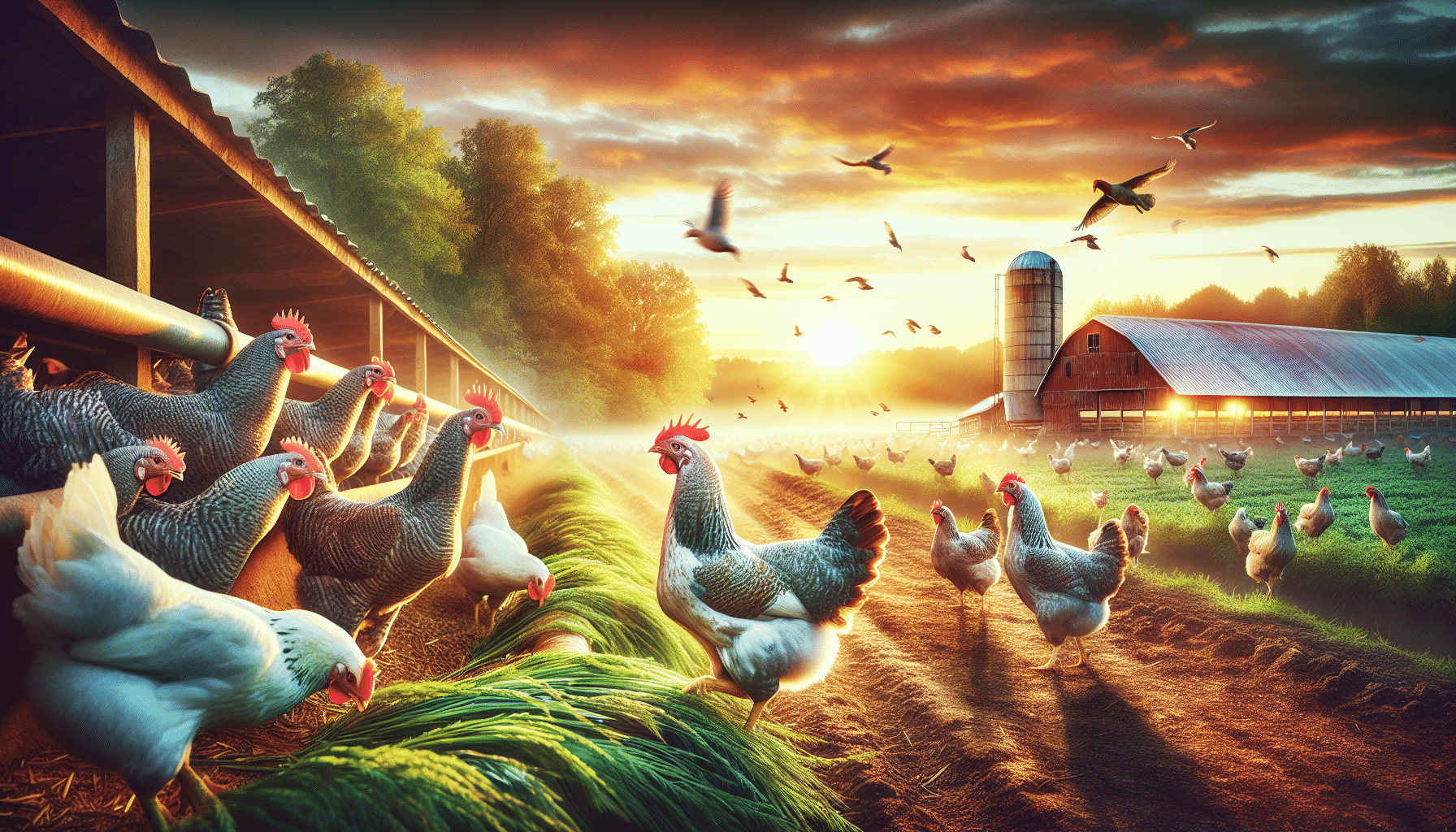This intricate drawing captures the early morning hustle on a farm as dawn breaks. Dominating the left side of the image, a variety of chickens are depicted near a long rectangular chicken coop adorned with a silver triangular roof. The chickens, in hues of pure white and distinctive black-and-white stripes, are bustling about, some pecking at grassy patches on the ground, while others peer out from silver metal poles running through the coop. Above, several birds, possibly geese or ducks, take flight against a sky painted in the warm colors of a rising sun, with golden yellows, oranges, and grays blending together amidst scattered clouds.

In the middle and extending towards the right, a large field carpeted with tall green grass hosts numerous chickens that appear to be grazing. A brown dirt road runs through the center of the scene, flanked by the active poultry. In the background, a classic red barn with a sharply contrasting silver silo stands tall, with trees framing the farmstead. This descriptive scene vividly showcases the daily activity of the farm, highlighting both the artistry of the depiction and the serene yet lively environment as the day begins.